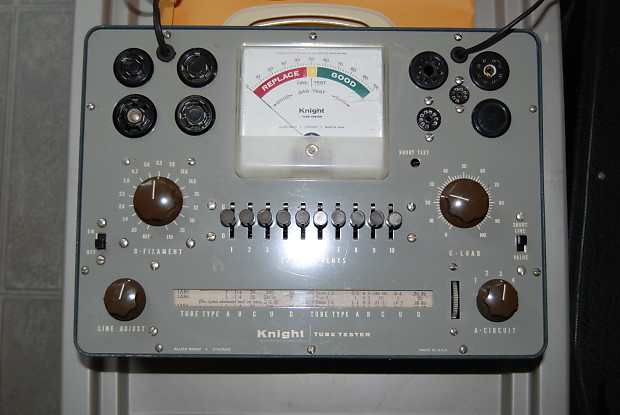The image depicts an old Knight Tube Tester, likely from the 60s or 70s, housed in a metallic gray box. The center features a prominent ammeter-like gauge with a white background, transitioning from red (labeled "replace"), through yellow, to green (labeled "good"). The gauge’s indicator currently points to "replace." Surrounding this gauge are various brown and black knobs with white indicator lines, numbers, and specific labels such as "line adjust" on the bottom left and "A circuit" on the bottom right. Additional text, including the company name "Knight" and the device title "Knight Tube Tester," is visible in white lettering at the bottom. The machine also includes switches and levers, with one switch labeled "on/off" positioned to the left. The device appears functional, allowing for cables to be plugged in, hinting at its use in testing electrical components.